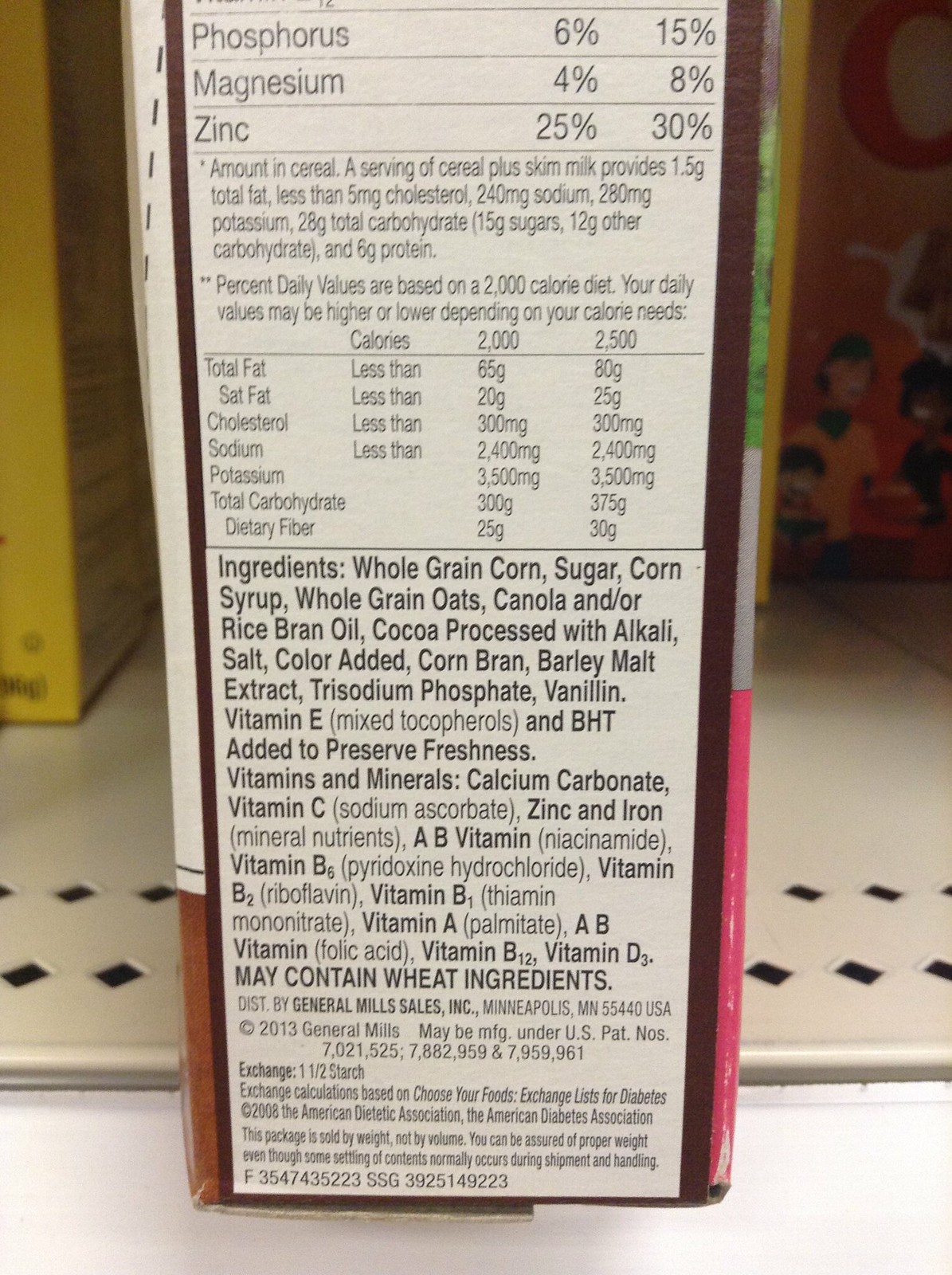The image depicts a close-up view of the side panel of a food box, likely a cereal or snack box, placed on a grocery shelf among other items. The visible portion of the box features a detailed nutrition facts section starting with phosphorus content listed as 6% and 15%, followed by magnesium at 4% and 8%, and zinc at 25% and 30%. The panel also includes an ingredients list, various warnings, a calorie chart, and the manufacturer’s copyright attributed to General Mills. Additionally, a patent number, the distributor's name, and the city and state of distribution are printed on the side. The image focuses on these details, providing a snippet of the box's comprehensive labeling.